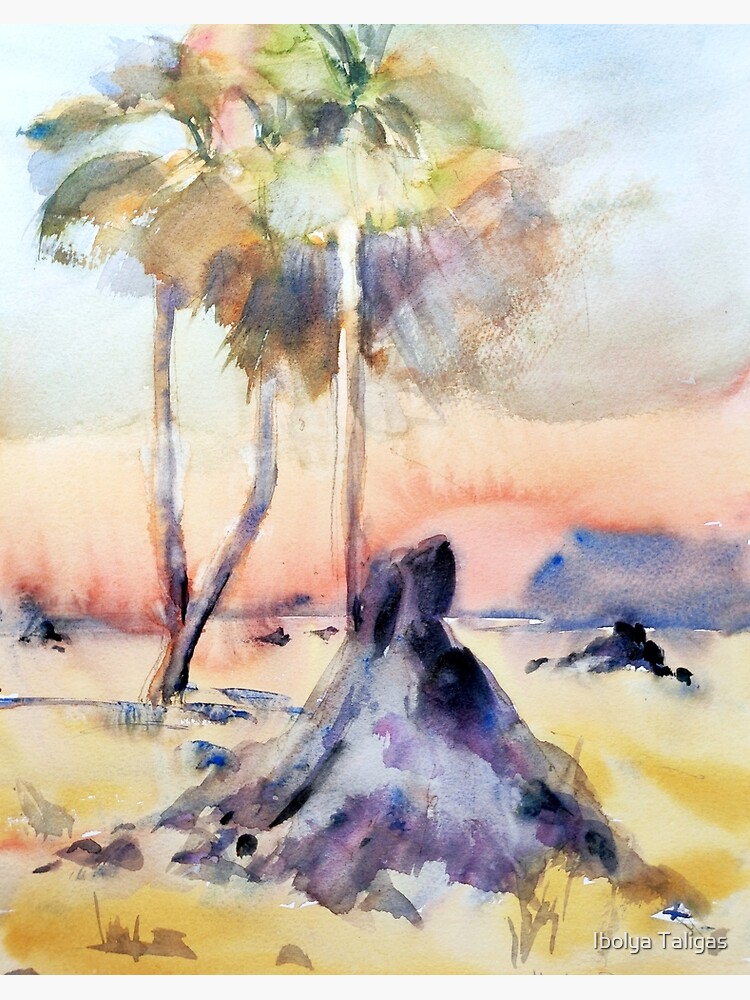The image is a rectangular watercolor painting with the artist's name, "Ibolya Taligas," inscribed in white font at the bottom. It presents a serene beach scene viewed horizontally. Dominating the background is a large palm tree with a distinctly brown trunk and leaves exhibiting mingling shades of green, brown, and pink. The foreground features a unique pyramid-shaped gray rock formation, akin to a small volcano, positioned in front of the tree on the yellow sandy beach. Above, the sky is layered with an abundance of white clouds and soft hints of blue at the top, transitioning to a pinkish hue near the horizon, indicative of a sunset. The sun appears halfway set, casting a warm glow over the scene. The painting's colors are vibrant and varied, including light blue, green, orange, purple, and gray, emphasizing the lively and bright setting.